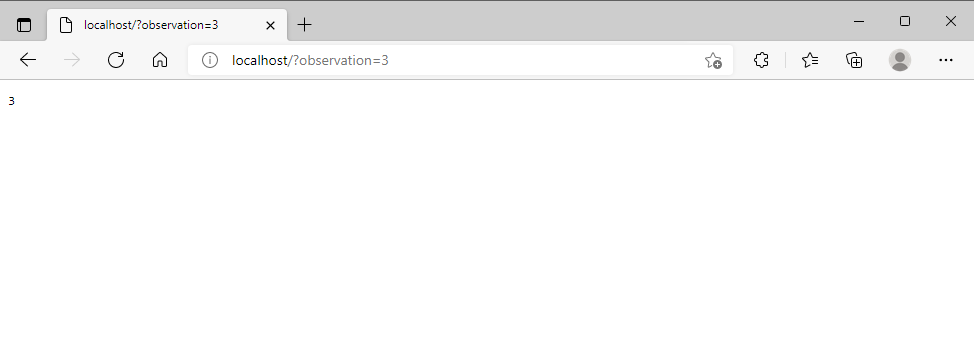This image showcases a web browser interface with a light gray border. At the top, there is an open tab displaying an icon on the left whose specifics are unclear. The tab text reads "localhost/?observation=3", and to the right of this text, there's an ‘X’ for closing the tab and a ‘+’ for adding a new tab. 

In the upper right-hand corner of the browser, there are three icons: a dropdown menu, a screen enlargement icon, and a close window icon. On the browser toolbar itself, you can find several navigation buttons. Progressing from left to right, there are a left-facing arrow for backward navigation, a right-facing arrow for forward navigation, a refresh icon to reload the page, and a home icon. 

The address bar in the middle features a small information icon preceding the URL "localhost/?observation=3." To the far right of the address bar, there is a star icon for bookmarking and a puzzle piece icon, likely for extensions. Additionally, there is a user's profile icon followed by three horizontal dots, indicating more options or settings.